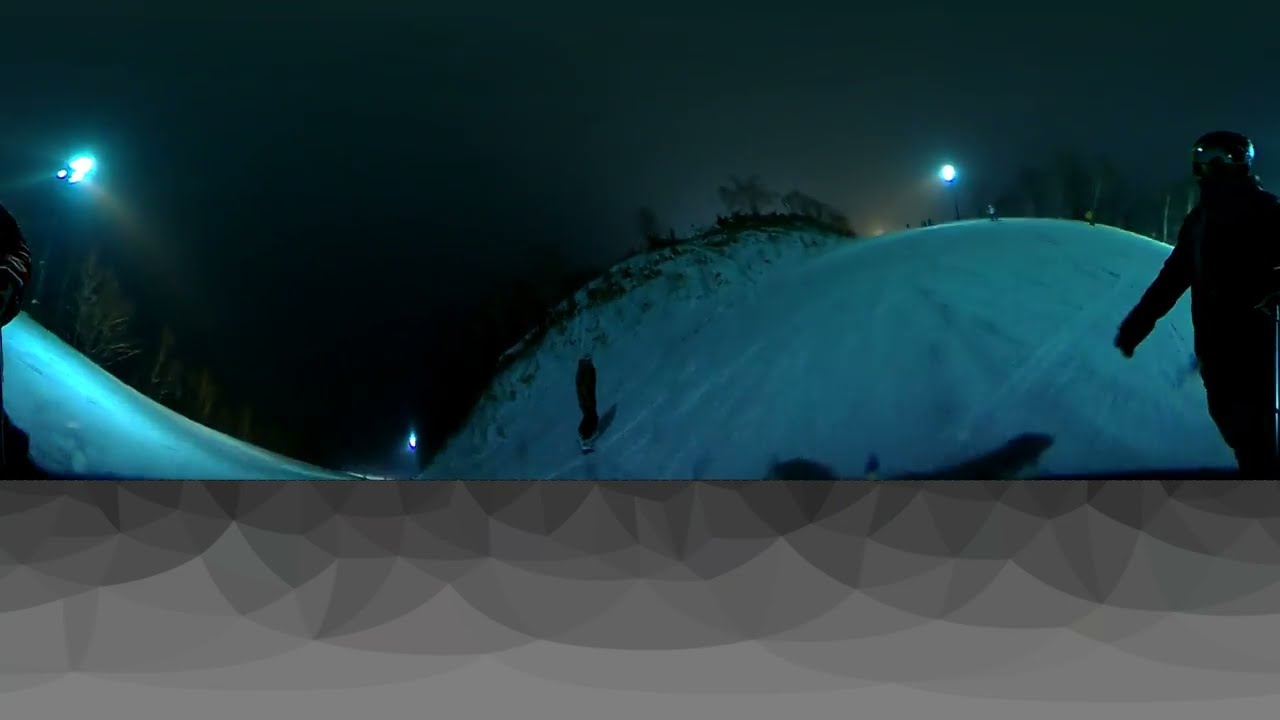The image captures a nighttime scene on a snowy ski hill. The top two-thirds of the image is a photograph showing the ski slope illuminated by scattered lights. Six skiers, dressed in various colored coats and snow pants (black, red, white), are navigating the slope. Notably, towards the very right-hand side, a skier wearing goggles, a mask, and a coat gazes towards the camera. In contrast, the bottom third of the image transitions from a photograph to a gradient of dark gray to light gray, adorned with abstract geometric shapes. The night sky overhead adds to the atmospheric ambiance of the snowy mountain scene.